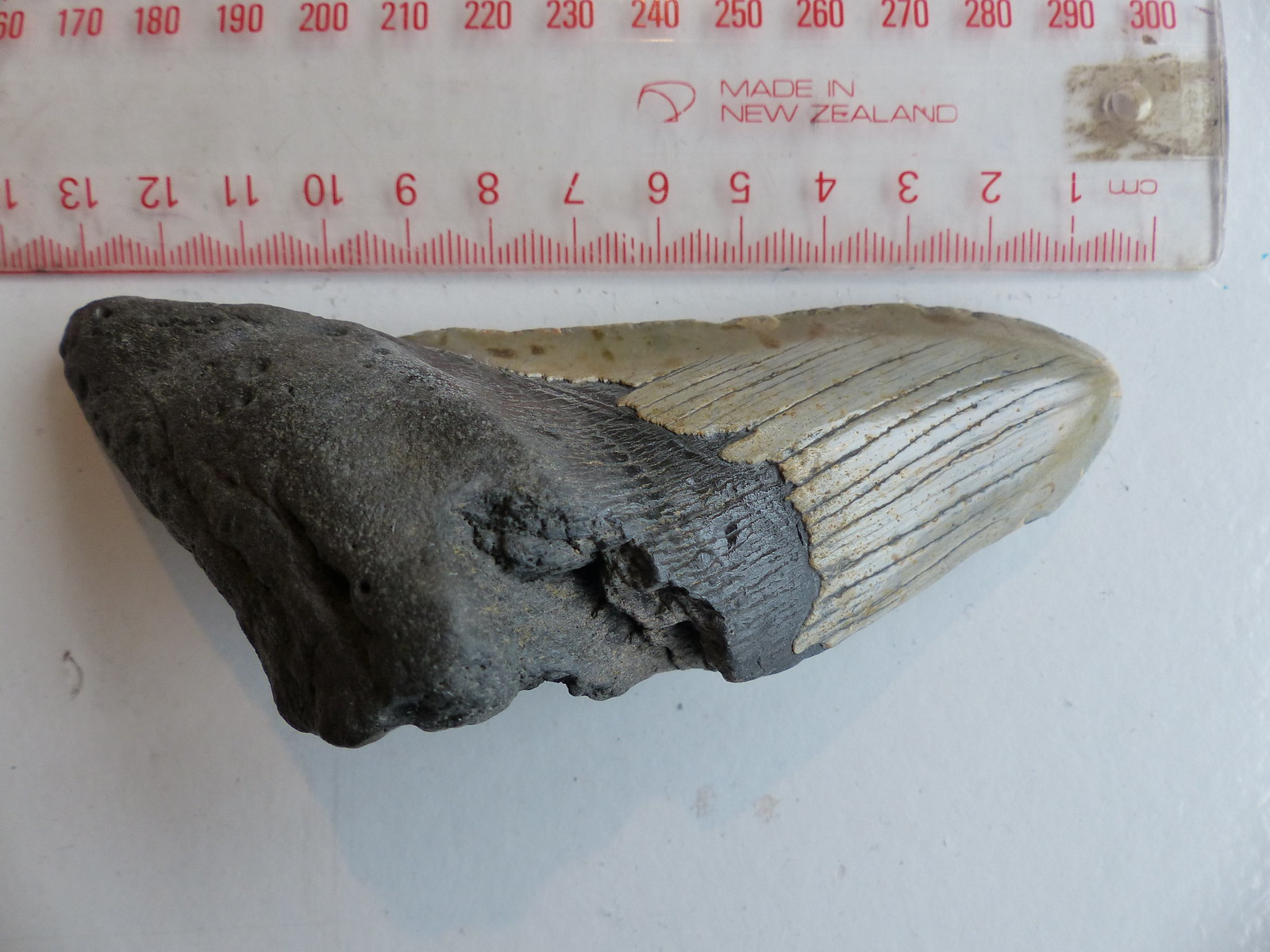The image depicts a large piece of fossilized bone, appearing to be a prehistoric animal tooth. The fossil is dual-toned, exhibiting a dark brown to almost black coloration on one side, and a silvery grey, white hue on the other. Positioned on a white table for a clear backdrop, a transparent ruler marked with red numbers is positioned directly above the fossil, measuring its length. The ruler is metric, showing measurements in centimeters and millimeters, ranging from 170 to 300 mm, and is made in New Zealand. The total length of the fossil is nearly 13 centimeters.